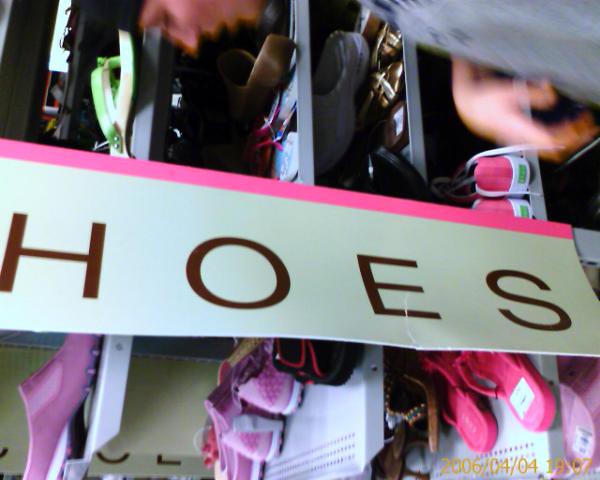This image, captured on a slightly rotated digital camera on 2006/04/04 at 19:07, depicts a display of various types of shoes arranged on grey shelves. The shelving is positioned both to the left and right of a fragmented sign. The sign has a green banner with brown letters, partially obscured to read "H-O-E-S," and features a pink stripe at the top. The shoes are mostly in shades of pink and red, with some black tennis shoes and sandals interspersed among them. A woman, identifiable by her hand and the grey shirt she is wearing, appears to be browsing the shoes. She also sports a black cap. The photo’s misalignment results in the person and the shoes appearing sideways. A green sandal is notably present at the top right corner of the image. The timestamp "2006-04-04" is clearly visible at the bottom right of the picture, although partially blurred.